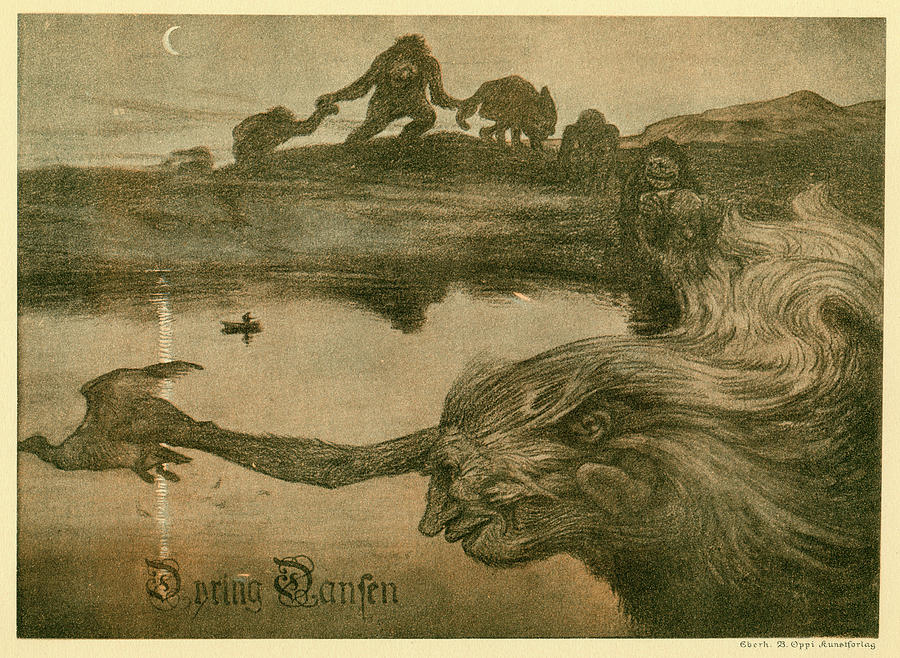This image is a detailed, grainy black and white drawing that appears to be done in a pencil sketch style. It depicts an outdoor night scene, framed by a light, almost flesh-colored border. In the upper right corner of the square image is a crescent moon with a yellow ridge. In the center of the image, there's a calm lake with slight ripples, and a small canoe with a lone figure paddling in the middle. Surrounding the lake, a row of various fantastical animals and mythological creatures create a circular pattern; some animals have interconnected limbs, and one creature on the left side reaches out to grab a bird, likely a duck or a goose, in the lower left corner. In the lower right corner of the border, there’s some indistinct lettering that is hard to decipher. Additionally, on the bottom edge of the image itself, there’s gothic-styled calligraphy that appears to spell out something akin to "Daring Danfin." The drawing includes the signature "G-Birth 21, Ops, Waffling" in the bottom right corner within the image.